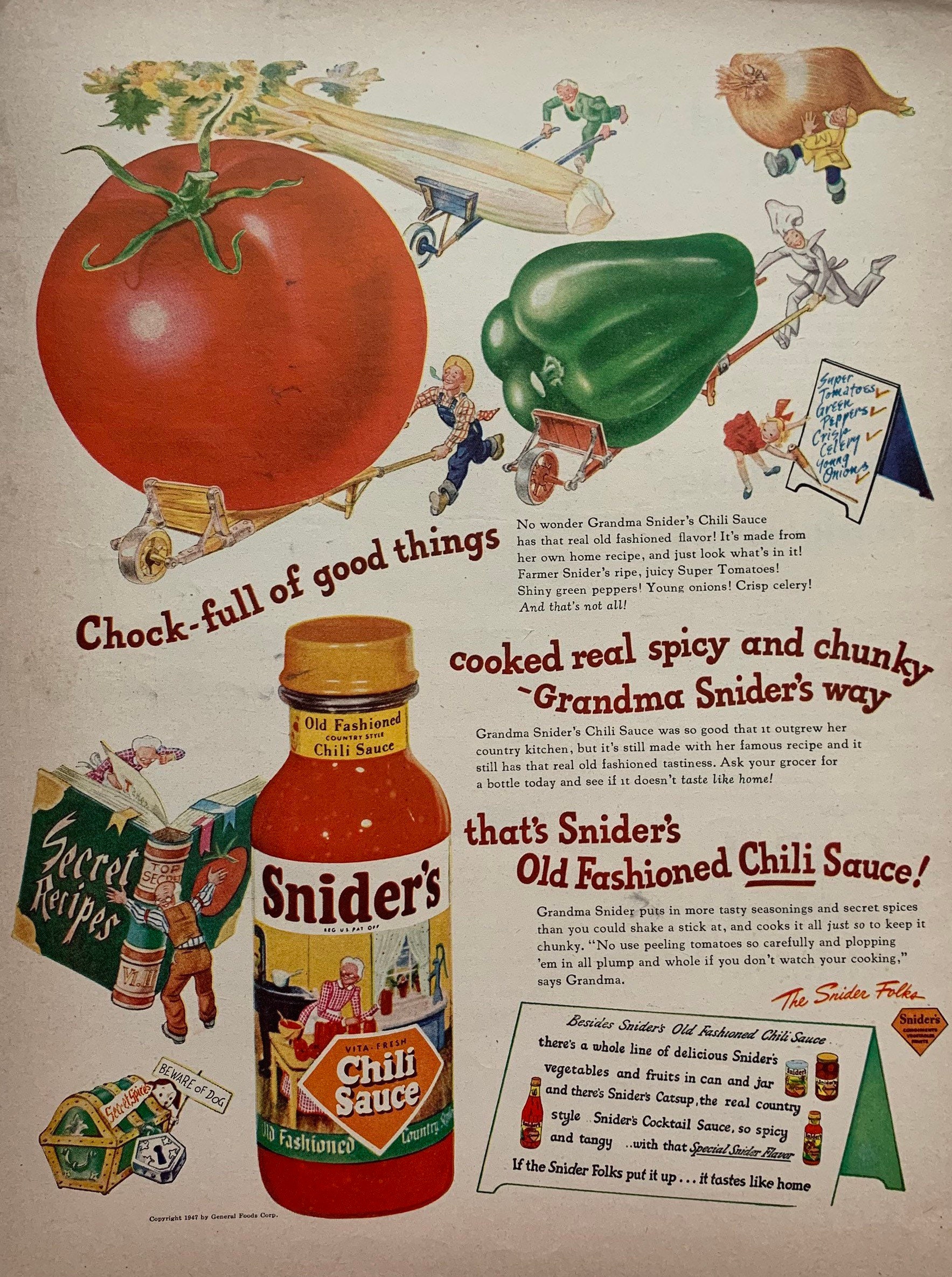This vintage full-page advertisement for Schneider's Chili Sauce is rich with intricate illustrations and vibrant colors. Dominating the top third of the dark brown paper poster are whimsical drawings of people, such as farmers, chefs, businessmen, and a sailor, all pushing oversized vegetables on dollies. The farmer on the bottom left pushes a giant ripe tomato, while the chef on the right is pushing a large green bell pepper. A businessman at the top maneuvers a huge stalk of celery, and the sailor in a yellow coat at the top right handles a large onion. 

Each character is detailed, with the farmer donning a straw hat and blue overalls, complete with a green straw piece in his mouth, and the chef dressed in a traditional white outfit. Surrounding these figures, scattered vegetables include a red tomato with a green stem, green celery, and a green bell pepper.

A playful little man carries a clove of garlic, while a woman in a red and white plaid dress and white apron appears to be jotting notes on a sign. There's a large opened green book labeled "Secret Recipes" being held by another figure, and a treasure chest, gold with silver locks, adds to the charm and mystery of the scene.

In large, wavy red text interspersed with smaller black text, the ad proudly touts: "Chock-full of good things, cooked real spicy and chunky, Grandma Schneider's way. That's Schneider's old-fashioned chili sauce." At the bottom left, a clear glass bottle of the chili sauce is prominently displayed with its red contents and yellow cap. The label features a detailed depiction of an elderly Grandma Schneider cooking in the kitchen, cutting red peppers on a wooden table against a yellow wall.

This elaborate and colorful advert engages viewers with its nostalgic charm and vivid depictions, effectively celebrating Schneider's old-fashioned chili sauce.